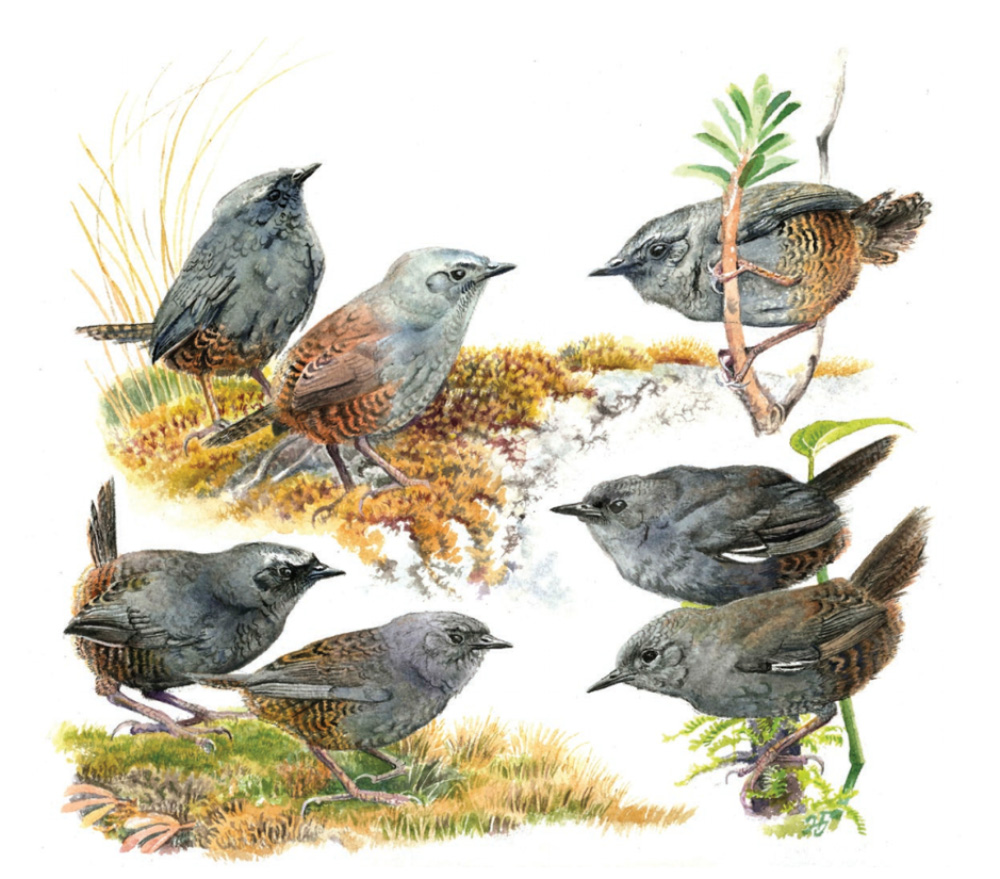The image is a detailed drawing of several birds resembling small finches with distinctive color patterns. The background is entirely white, contrasting with the artfully rendered birds. Each bird exhibits a predominantly grey plumage that transitions into a striking orange and black tiger stripe pattern on their tails and back legs. In the top left of the drawing, two birds—one darker grey and the other lighter grey—are positioned side by side, both gazing towards the right. The top right features a single bird perched gracefully on a branch, looking to the left. At the bottom left, two dark grey birds are depicted on the ground amidst a patch of grass. Meanwhile, on the right, two similarly patterned birds are perched together on another branch. The scene is enriched with additional details like grass and wheat-colored stems emerging from the hand-drawn earth, enhancing the naturalistic feel of the illustration.